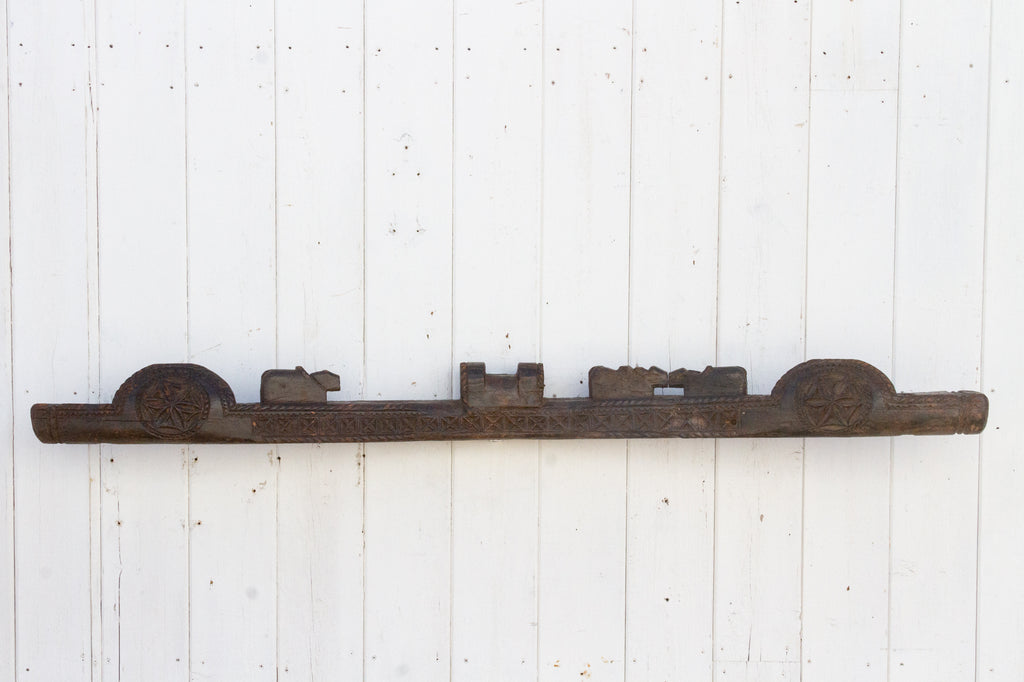The photograph appears to be taken outside, capturing an intricate scene. The image showcases a white wall made up of vertical wooden planks painted in white. The wooden surface features numerous nail holes concentrated at the top and bottom edges, adding a weathered texture to the backdrop. Attached to this rustic wooden wall is a long wrought iron pole, possibly resembling an old car axle. This metal piece displays a pattern with two small bumps at the top and three rectangular shapes of differing sizes between these bumps, adding to its antique appearance. Additional detail includes what looks like carvings or shapes on the pole, and to the right, two small wooden cow figures seem to be part of the scene, further enriching the visual complexity of this unassuming yet detailed composition.